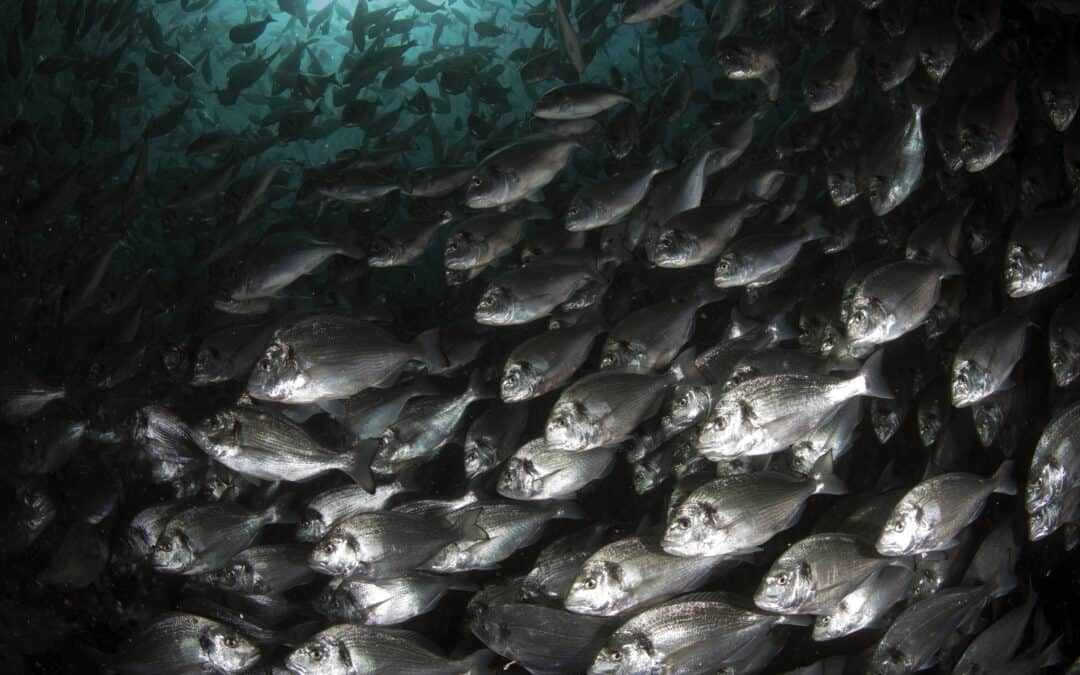This image is an underwater photograph showcasing a very large school of small, silver fish in a deep, turquoise blue sea. In the foreground, a densely packed formation of hundreds of these shiny, medium-sized fish, each with rounded bodies, short side fins, and short tail fins, swim uniformly from right to left. Their collective movement seems to form a protective mechanism against predators, indicating the principle of safety in numbers. Against the tranquil blue backdrop, more fish are visible, swimming randomly in various directions, suggesting the possible presence of predators nearby. At the top left, sunlight breaks through the ocean surface, casting an ethereal glow. In the distant background, there appear to be other indistinct sea creatures, perhaps jellyfish, adding to the mystique of the deep sea scene.